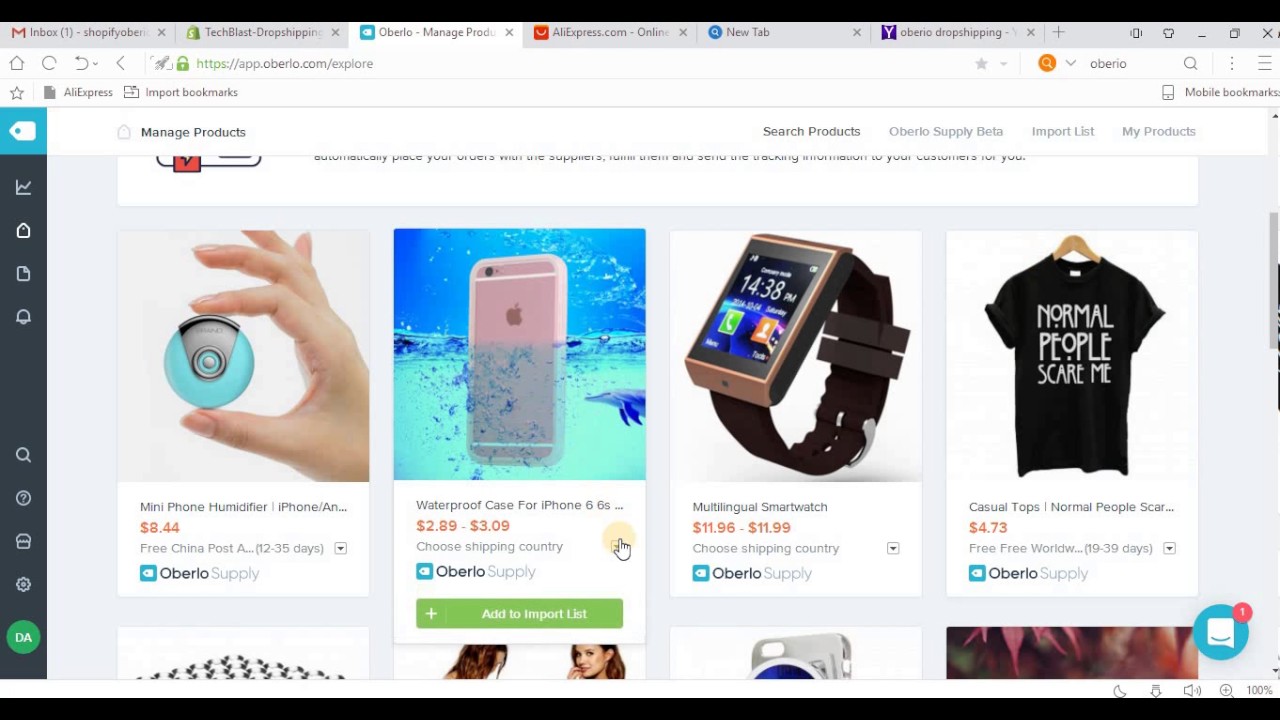The screenshot captures a web page viewed on a computer. At the very top of the page is a long, black rectangular bar. Below this bar are several gray rectangular tabs, each containing text. The first tab reads "Inbox (1)," the second tab says "Technological Depot Shipping," followed by "Manage Products," "aliexpress.com," "New Tab," and "Shopping."

Underneath the "Manage Products" section, various product listings are displayed with images and descriptions. A person's hand holds a small blue item labeled "Mini Phone Humidifier for iPhone" priced at $8.44. Another image shows a cell phone submerged in water with a small dolphin swimming nearby, advertising a "Waterproof Case for iPhone" priced between $2.89 and $3.09, offered by OBERIO supply, indicated by a blue square beside it.

Further down, an image of a "Multilingual Smartwatch" is shown with a price range of $11.98 to $11.99, also from OBERIO supply. Lastly, a black t-shirt with the text "Normal People Scare Me" printed in white on the front is listed for $4.73.